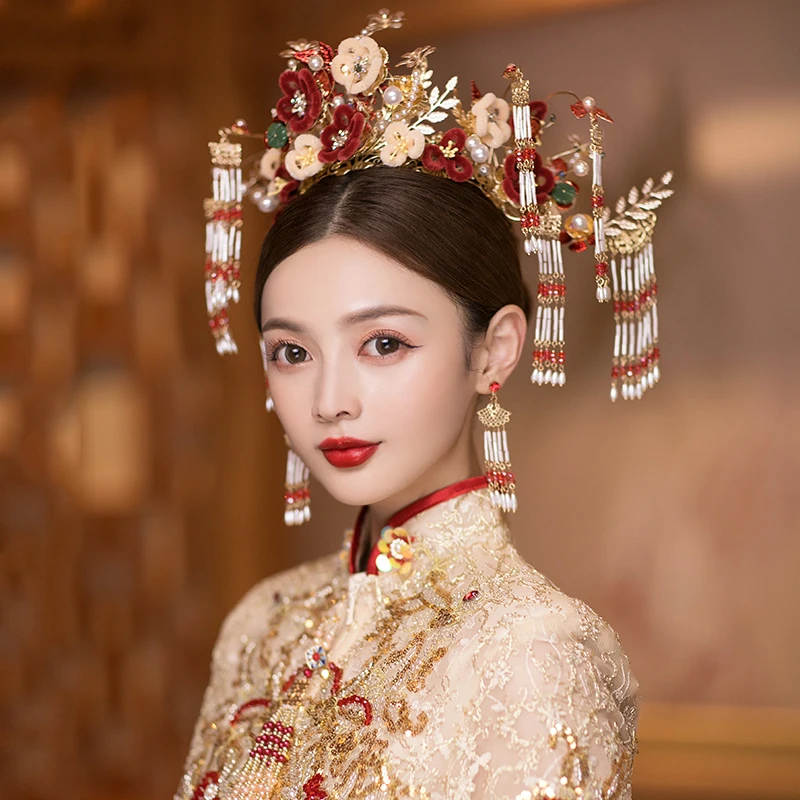This image portrays a young Asian female model adorned in a resplendent, traditional Chinese royal outfit. Her dark brown hair is elegantly styled to showcase an ornate headdress, reminiscent of ancient Chinese royalty, featuring white and red handcrafted flowers made of felt-like material and stems with leaves, all interspersed with pearls. This intricate headpiece extends to include dangling beaded jewelry, similar to decorations found on Native American dream catchers. These beads also complement her matching earrings, which hang elegantly from a gold, pretzel-shaped design.

Her makeup is striking, with bold red lipstick, large eyes accentuated with cat-eye styled eyeliner, and subtle eyeshadow, giving her a regal, yet contemporary look. The elaborate dress she wears is a vision of yellow silk adorned with intricate gold and red beadwork, including a high collar that reaches her neck, adding to the garment's historical allure.

The photograph appears to be taken in a professional setting, with a blurred background and bright, even lighting that illuminates her face, emphasizing her poised and elegant demeanor. The overall composition suggests she is likely modeling this traditional attire, showcasing its ornate beauty and cultural significance.